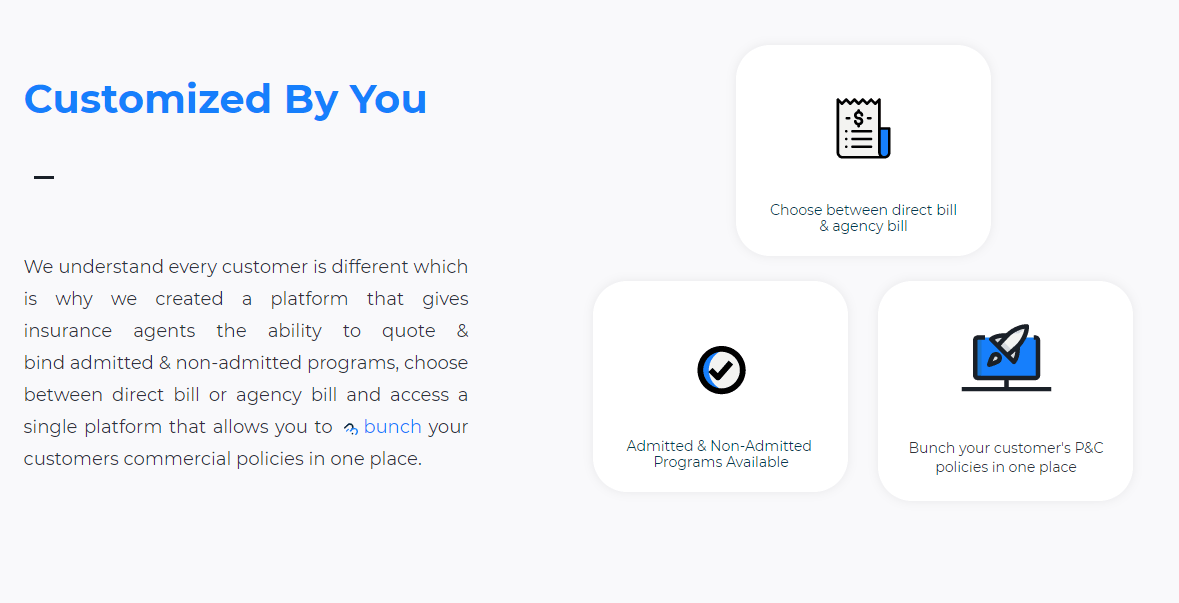The image features a window with a prominent title in bold blue text that reads "Customized by You." Below this title, there's a paragraph of black text explaining the concept. The text reads: "We understand every customer is different, which is why we created a platform that gives insurance agents the ability to quote and bind admitted and non-admitted programs. Choose between direct bill or agency bill and access a single platform that allows you to consolidate your customers' commercial policies in one place."

Within the window, there are three boxes arranged in a triangular formation, each containing an infographic detailing specific features. 

1. The top box is labeled, "Choose between direct bill and agency bill," and includes an icon of a receipt.
2. The bottom-left box reads, "Admitted and non-admitted programs available," accompanied by a black circle with a tick inside.
3. The bottom-right box states, "Consolidate your customers' P&C policies in one place," depicted by an infographic of a rocket inside a computer monitor.